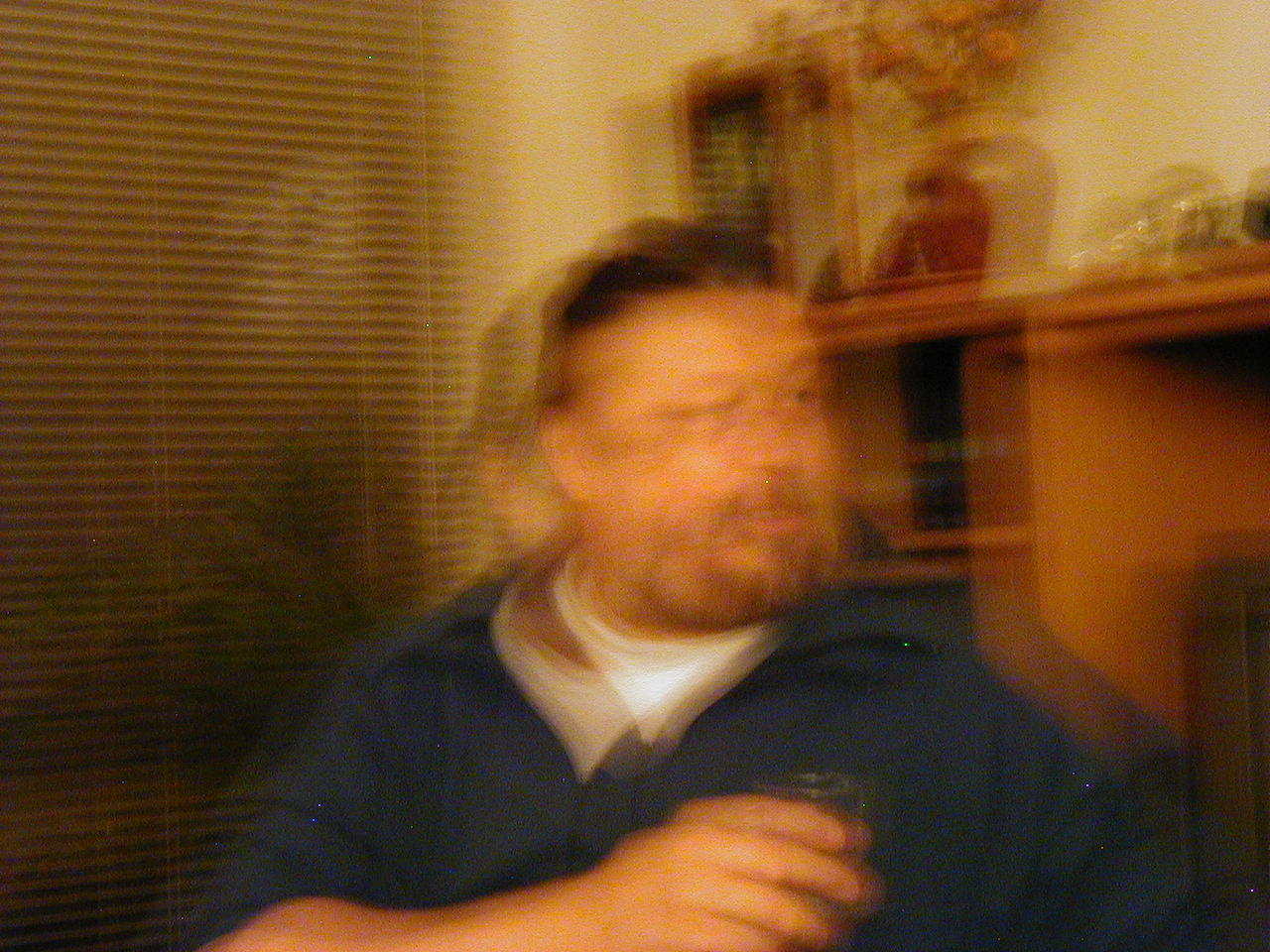This image captures a man in a dark blue short-sleeved shirt over a white t-shirt, holding a small glass, possibly a shot glass, in his right hand. His hair is slicked back and he sports a mustache and a goatee. The photograph appears double-exposed, resulting in a blurry, doubled effect where the man's features, as well as the background elements, are duplicated. The scene takes place indoors, revealing a yellowish-pink wall with an entertainment unit made of medium-colored wood behind the man. On the unit's shelves, there seems to be a vase with flowers and some indistinct items. To the left, a window with Venetian or bamboo blinds partially reveals some greenery outside, possibly a bush. The overall yellowing of the film adds to the aged look of the photograph.